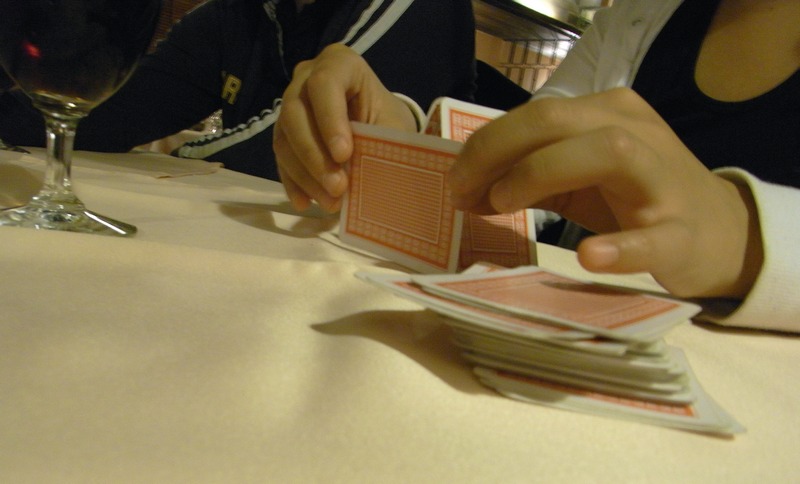The image depicts a table draped in a lemon-yellow or butter-colored fabric. At the center of the table, there is a wine glass, though it's unclear if it contains any liquid. Seated closely side by side around the table are two individuals, visible only from the neck to the chest as they lean forward. The person on the left is wearing a black zip-up sweater with white stripes along the sleeves. The individual on the right is dressed in a black inner blouse paired with a white jacket. This person is engaged in an activity involving playing cards. The cards are arranged in a stack, face down on the table, with three additional cards laid out in front of the individual. The person is holding one of these cards horizontally between their fingers, leaving the identity of the cards a mystery.